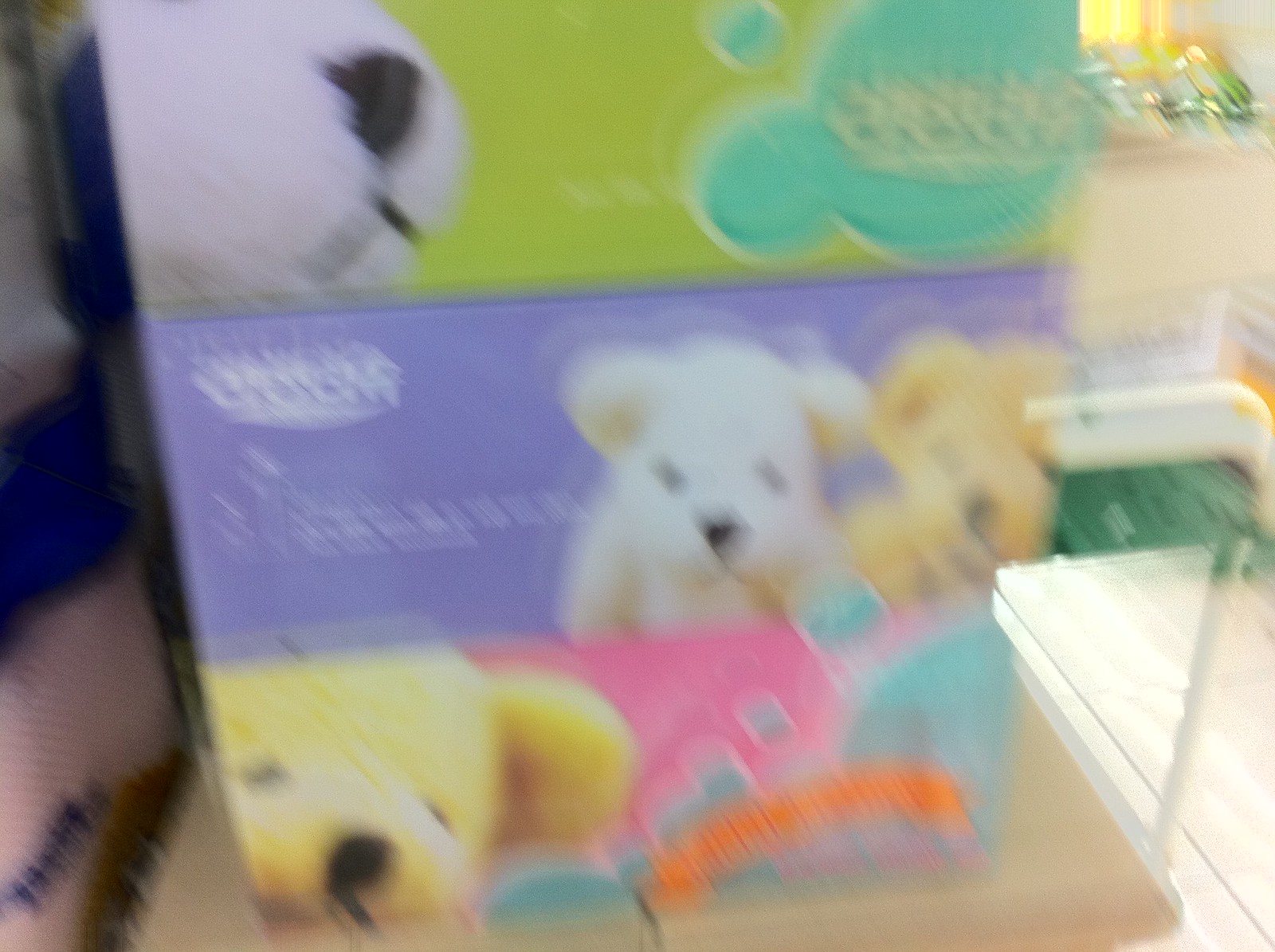This blurred photograph depicts a collection of cardboard boxes featuring images of stuffed bears, situated on a light-colored wooden floor. The boxes are stacked on a chair with a tan-colored seat and metallic white arms. Sunlight streams in from a window in the upper right-hand corner, casting a warm light over the scene. 

The bottom box, with a bluish-purple hue, showcases three bears: a prominent white bear with black eyes and a black nose in the middle, flanked by yellowish-brown bears. This box also features an unreadable text and various shapes, including a pink house-like figure with an orange band.

Above it, a lavender box displays a white bear on the left and a golden-yellow bear to the right. Crowning the stack is a box with a yellow-green background, depicting a close-up of a stuffed bear's snout and nose, alongside greenish-blue bubble shapes on the right. 

The overall image is streaked and blurry, likely due to camera motion, and hints at additional background elements like a window and possibly a countertop or sink area, though these details are indistinct.